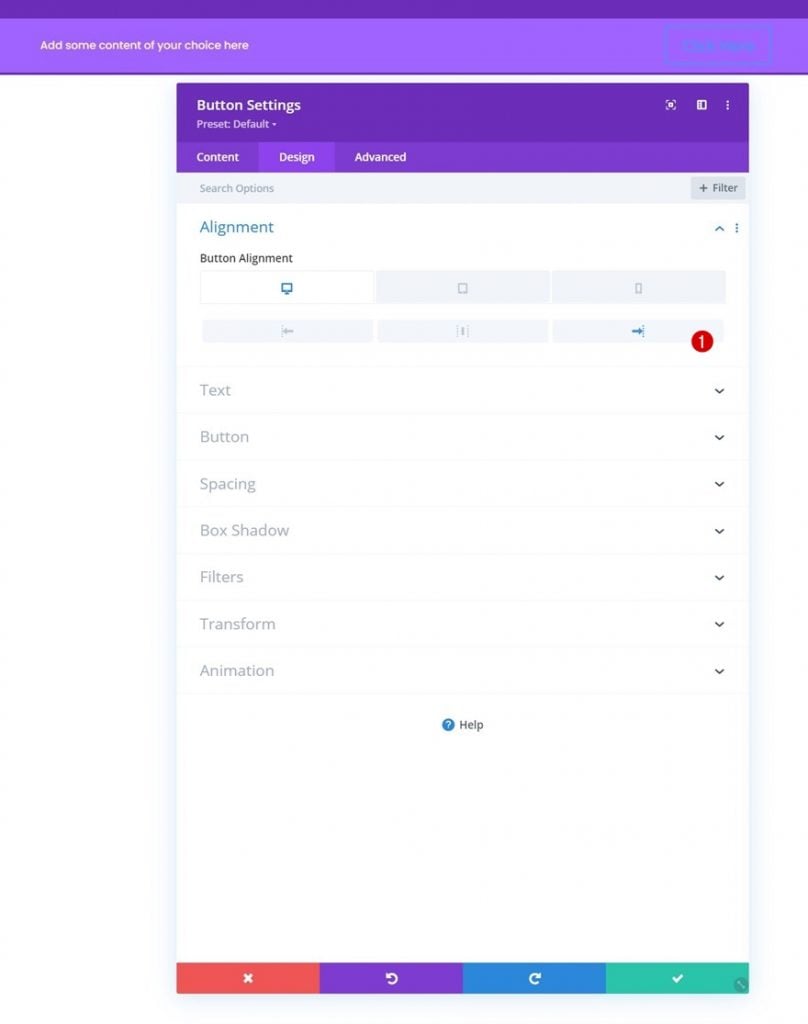The image displays a website interface featuring a prominent, two-toned purple banner at the top. The uppermost section of the banner is a dark purple, transitioning into a lighter purple below, which contains the placeholder text: "Add some context, add some content of your choice here." On the right side of this light purple section, there is a blue square or rectangle with unreadable text inside.

Beneath the banner, the website background is primarily white. A vertical rectangular section on the site includes a dark purple header labeled "Button Settings." This header features a drop-down menu set to "preset default" with an accompanying down arrow. Below this, the interface has three tabs: "Content," "Design," and "Advanced," with the "Design" tab currently selected.

The "Design" tab reveals various customization options:
- A section titled "Search Options" with a rectangular input area.
- An "Alignment" section for "Button Alignment," displaying icons of a computer, a square, and a cell phone. It also includes left, center, and right alignment arrows.
- Further customization options listed as "Text," "Button," "Spacing," "Box Shadow," "Filters," "Transform," and "Animation."

Adjacent to the right alignment arrow, there is a small red circular notification icon with the number one inside. On the right side of the interface, there is also a visible drop-down menu.

Overall, the interface appears to be a detailed, customizable design page for editing website buttons and related layout settings.